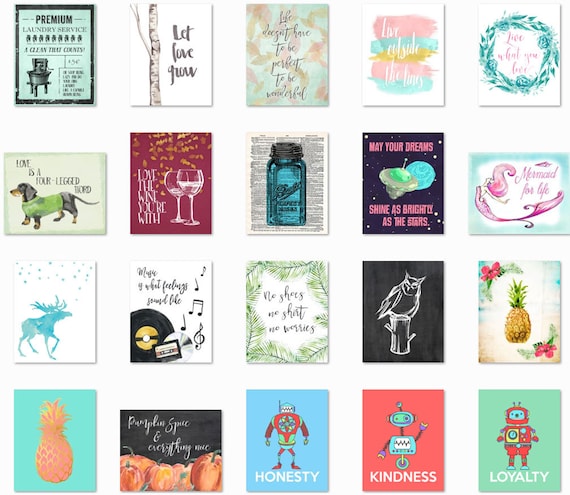The screenshot features an array of 20 distinct cards arranged in a 4x5 grid. Each card displays different text or imagery, contributing to a diverse collection. The first card's text is too detailed to read clearly. The second card reads "Let love grow." One of the cards in the first row states, "Life doesn't have to ..." though the rest of the text is unclear. On the second row, one card depicts a wiener dog. Beside it, there is a card featuring a couple of glasses of wine. The third row includes a card with a moose, another with a record adorned with musical notes, and additional cards showcasing a pineapple and an owl, respectively.